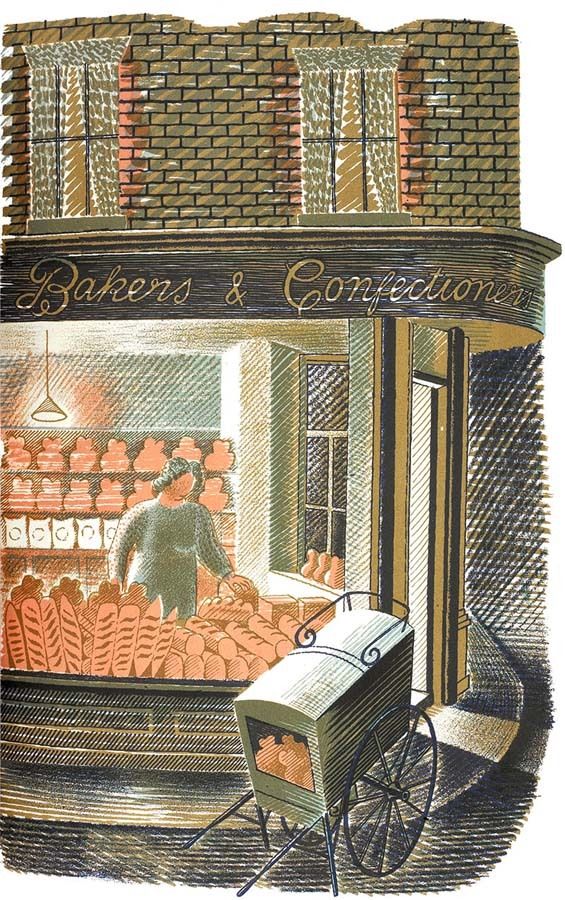This image, rendered in a cartoon or digital painting style, depicts an outdoor setting in front of a bakery store with the sign "Bakers and Confectioners" prominently displayed at the top in dark brass metal. The storefront is situated on the corner of a building with a blackish gold brick façade featuring two closed windows with partially open curtains, suggesting residential apartments above.

The scene takes place at nighttime, adding a darker ambiance to the setting. Below the sign, a large storefront window allows a glimpse into the bakery, where a woman with black hair, dressed in an olive green or gray dress, is seen looking down at various baked goods, including loaves of bread and possibly cookies arranged on shelves behind her. These shelves are softly colored, featuring packages and food containers, and are illuminated by a single hanging light with a triangular shade. To the right of the woman, there is a door suggesting an entrance to the bakery.

In front of the door stands a vendor's cart, painted in light green and resembling a wheelbarrow with handles and a single wheel. The cart is filled with brown packages, potentially containing bread or other baked goods. The overall aesthetic of the image combines a nostalgic, timeless feel with the detailed, warm charm of a small-town bakery at night.